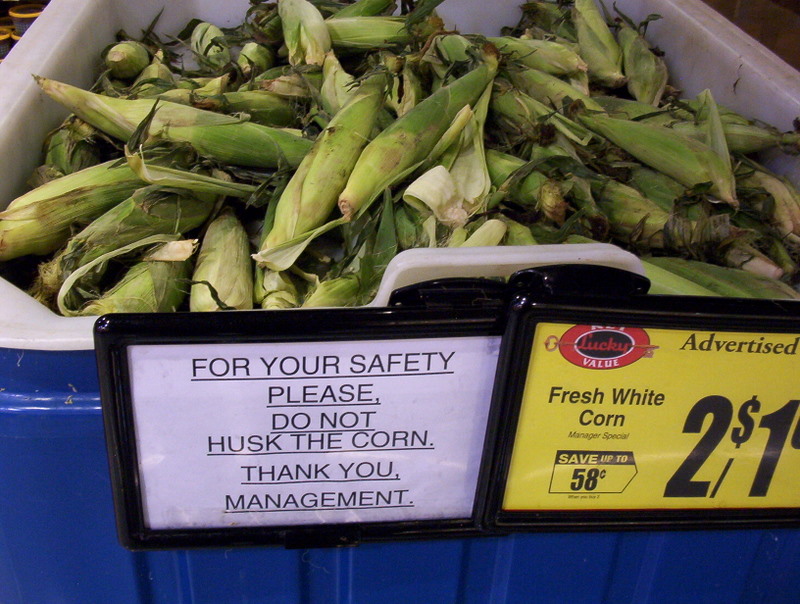In this color photograph, a large blue bin with a white interior is filled to the brim with unshucked ears of corn, their green husks hinting at their freshness. The bin is situated in what appears to be an outdoor market or grocery store setting. The top half of the image showcases the piled corn, while the bottom half displays the front of the bin and two attached signs.

The sign on the left, framed in black plastic, features a white background with black text that reads: "For your safety, please do not husk the corn. Thank you, Management," all underlined. The right sign, also bordered in black, is yellow with black text. It includes a red elliptical logo on the top left that reads "Lucky Value." Next to the logo, the word "Advertised" is printed, followed by "Fresh White Corn." Below this notice, the cut-off price indicates "2 for $1," with small text mentioning savings up to $0.58. The setting and meticulous signage add a layer of structured realism to the photo, emphasizing the vibrant and fresh appeal of the corn on display.